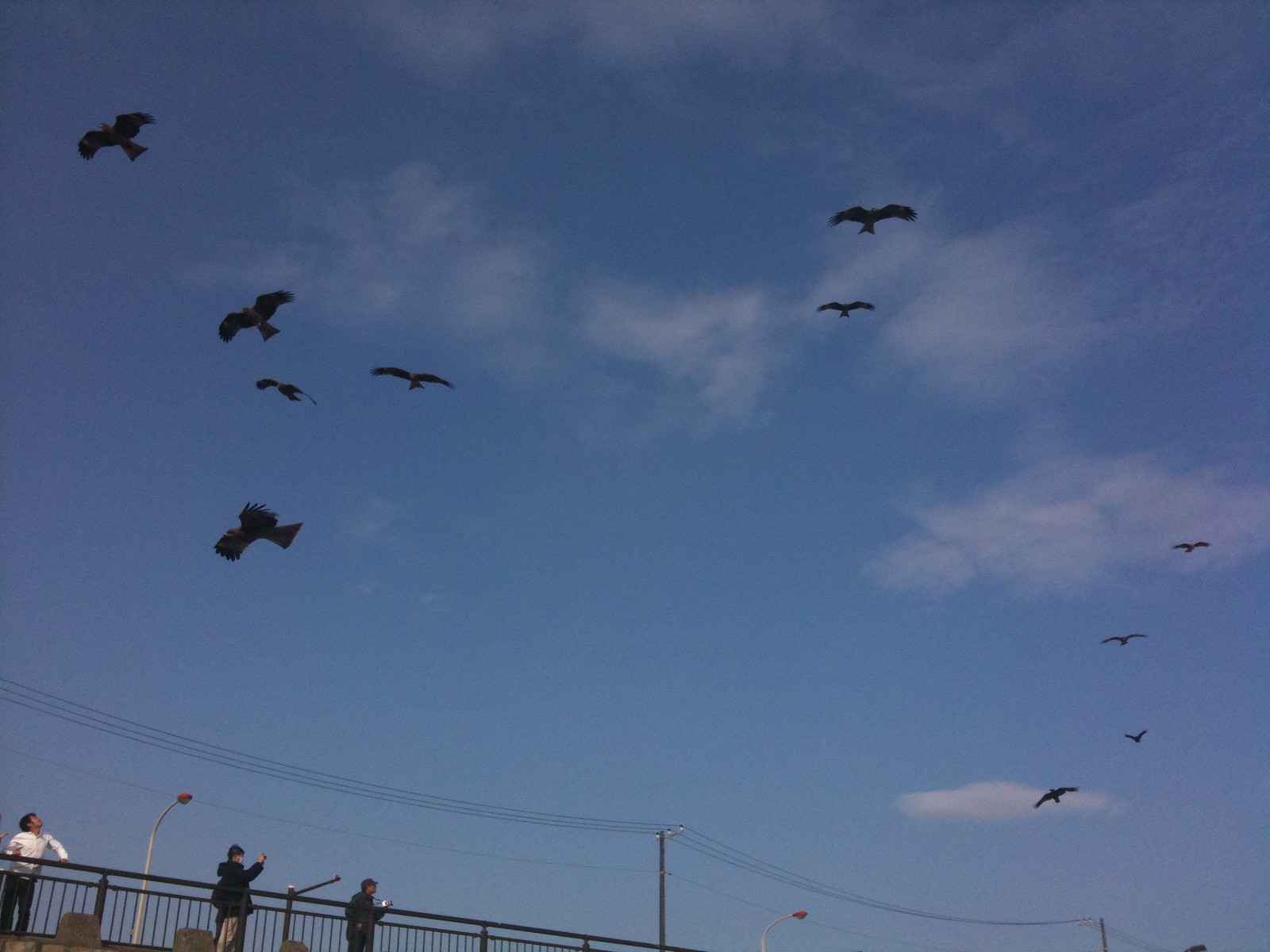The photograph is a horizontal rectangular image capturing a predominantly clear, deep blue sky with some faint, translucent white clouds scattered high above. The main focus of this image is a flock of eleven birds, all black silhouettes, gliding across the sky in various formations. These birds, possibly predator birds like eagles or hawks, are spread across the left to center and lower right parts of the image. 

In the bottom left corner of the photograph, three people are standing on a dark-colored overpass or side rail made of a metal top with vertical bars underneath. The people, detailed with dark and light clothing and one person pointing up, are all looking towards the sky, seemingly captivated by the birds above. Additionally, there are three parallel telephone wires running horizontally in the middle of the scene intersected by poles, while silver street lights with red tops are visible as well.